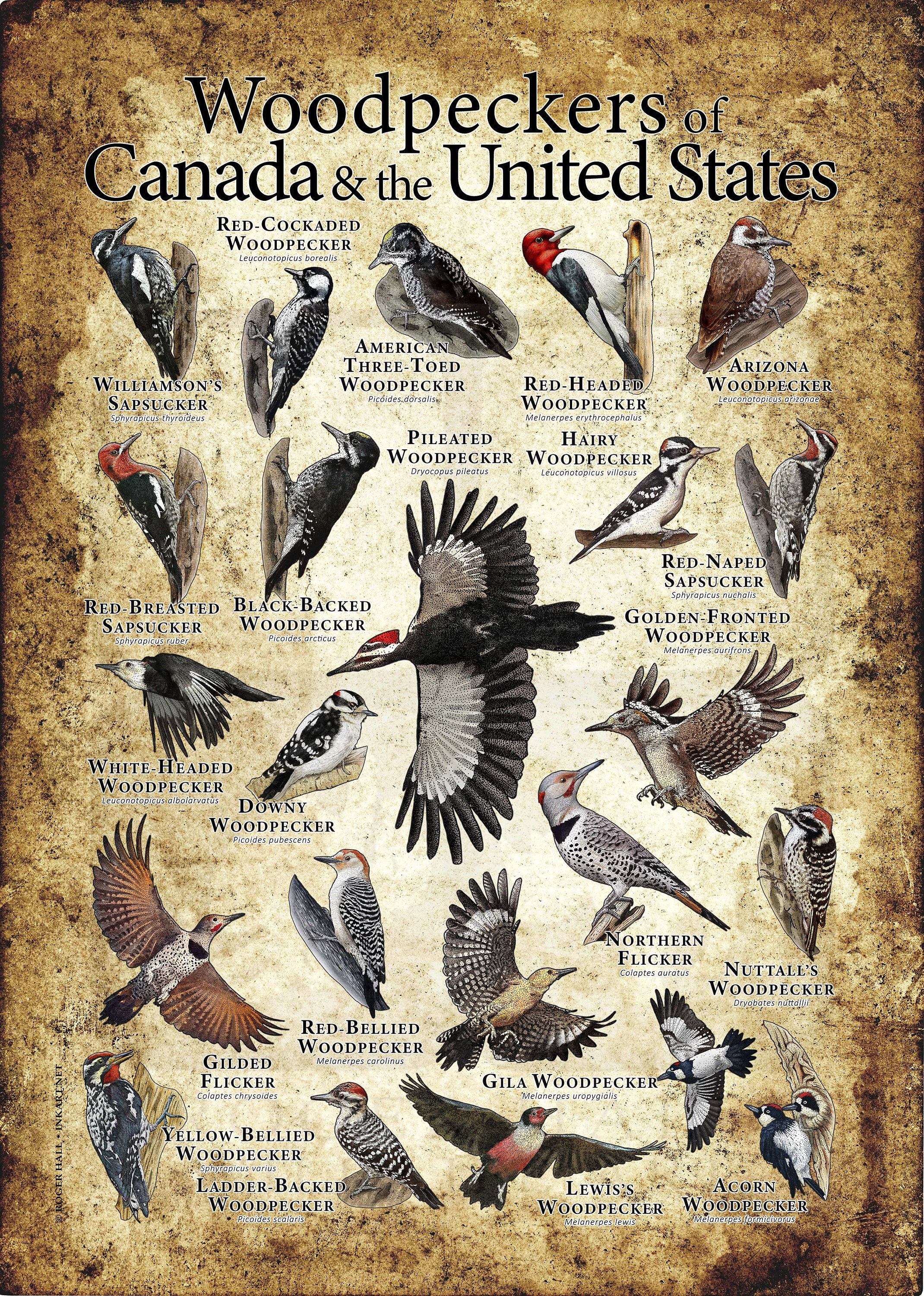The image is a vertical rectangular poster showcasing various species of woodpeckers found in Canada and the United States. The background features a textured gradient that transitions from a dark brown at the edges to a lighter beige or cream color in the center, complemented by subtle black speckles. At the top, bold black text reads "Woodpeckers of Canada and the United States." 

The poster displays numerous images of different woodpeckers, each carefully labeled with their names in black text. The birds are arranged within the lighter central area of the poster, ensuring each species stands out clearly against the contrasting background. Among the woodpeckers depicted are Williamson's sapsucker, red-cockaded woodpecker, American three-toed woodpecker, red-headed woodpecker, Arizona woodpecker, red-breasted sapsucker, black-backed woodpecker, pileated woodpecker, hairy woodpecker, red-naped sapsucker, golden-fronted woodpecker, white-headed woodpecker, downy woodpecker, northern flicker, Nuttall's woodpecker, acorn woodpecker, Lewis's woodpecker, Gila woodpecker, red-bellied woodpecker, gilded flicker, yellow-bellied woodpecker, and ladder-backed woodpecker. The images may also include brief descriptions, possibly with Latin names, adding scientific context to the visual display.